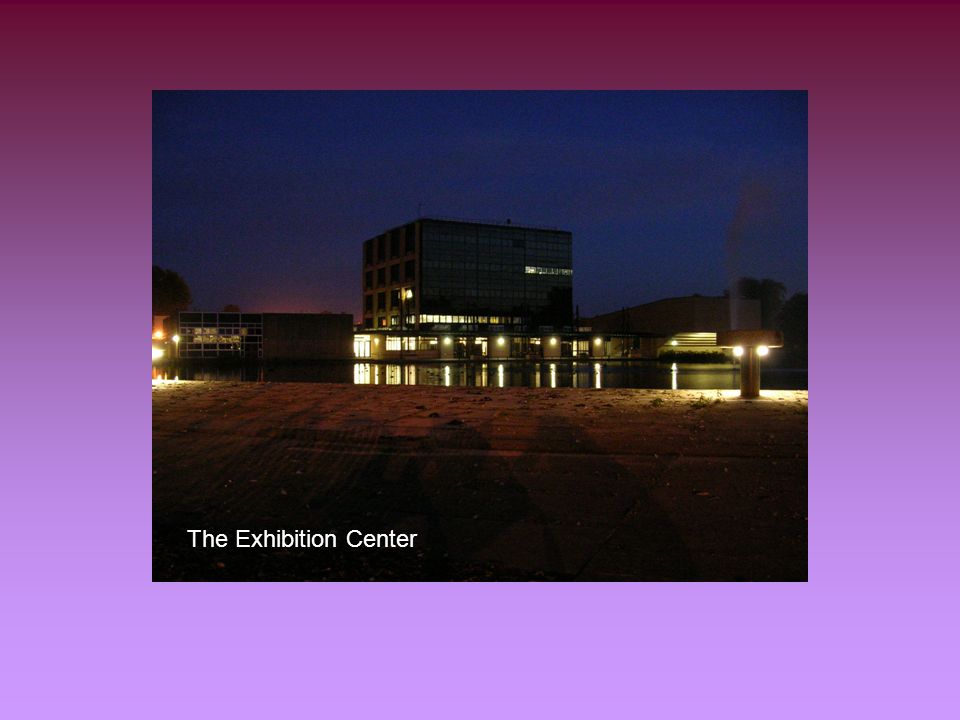The horizontal, rectangular image prominently features a nighttime scene with a row of buildings at the center, flanked by a decorative border that transitions from a dark magenta-purple at the top to a lighter violet-purple at the bottom. The photograph captures a three-building complex: a central, six-story building with dimly lit windows and adjacent two-story buildings on both the left and right, also sparsely illuminated. Each of the partial side buildings has very bright lights. The dark blue sky serves as the backdrop, creating a stark contrast against the sporadically glowing windows. In the foreground, a large open area resembling a mix of dirt and sand stretches out toward what appears to be a small moat or lake. In the bottom left corner of the image, in small white font, is the label "The Exhibition Center," while in the bottom right corner, the same inscription is also visible. The dim lighting and the setup give a sense of serene isolation, highlighted by the central building's unreadable sign and two well-lit posts in the yard.